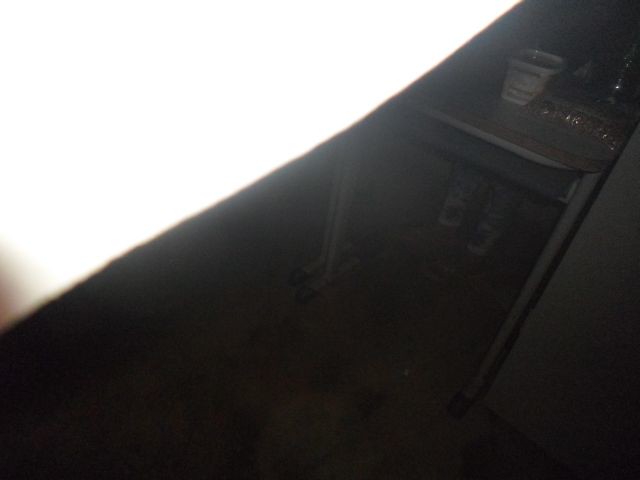This image features an undefined black object occupying the right side of the frame, with a potential hook or enclosed section visible at the top-right corner. The object's details are obscured by its dark coloration, making it challenging to identify. Contrasting with the object, the upper-left background is a stark white, emphasizing the object's silhouette. The ambiguous nature of the dark item, which could possibly be a suitcase or another type of container, adds an element of mystery to the scene due to insufficient visual information.